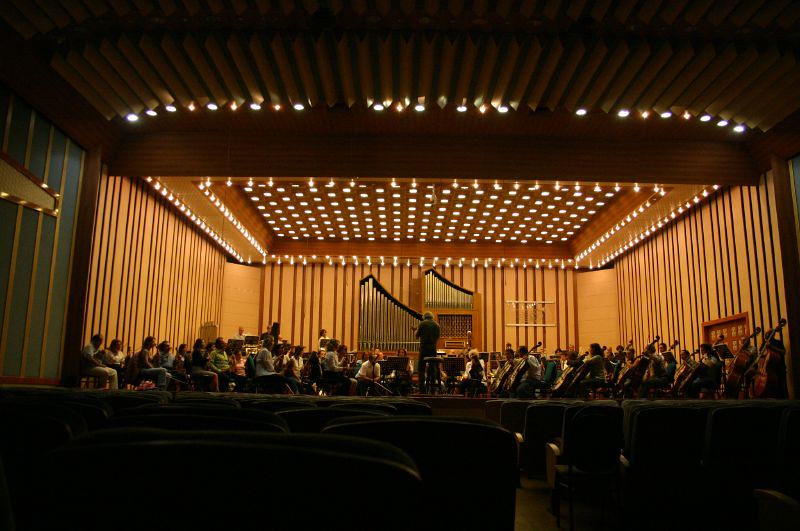The image depicts an illuminated concert hall, showcasing a classical orchestra amidst a rehearsal. The stage, elevated about five feet above the seating area, features wooden-framed walls and ceiling, adorned with numerous lights. The right side of the stage is occupied by several rows of cellists, with three upright bass players visible in the back. Adjacent to the cellists are sections for violinists and brass players. A central figure dressed in black, presumably the conductor, addresses the orchestra. A striking metal organ stands prominently in the background alongside kettledrums. The seating area for the audience is entirely empty, emphasizing the rehearsal nature of the setting. The people in the orchestra are too distant to determine specific ages, making it ambiguous if this is a high school or a professional group. Colors in the image span shades of black, white, gray, brown, blue, green, and red. The overall ambiance conveys a detailed and vibrant preparation for an upcoming performance.